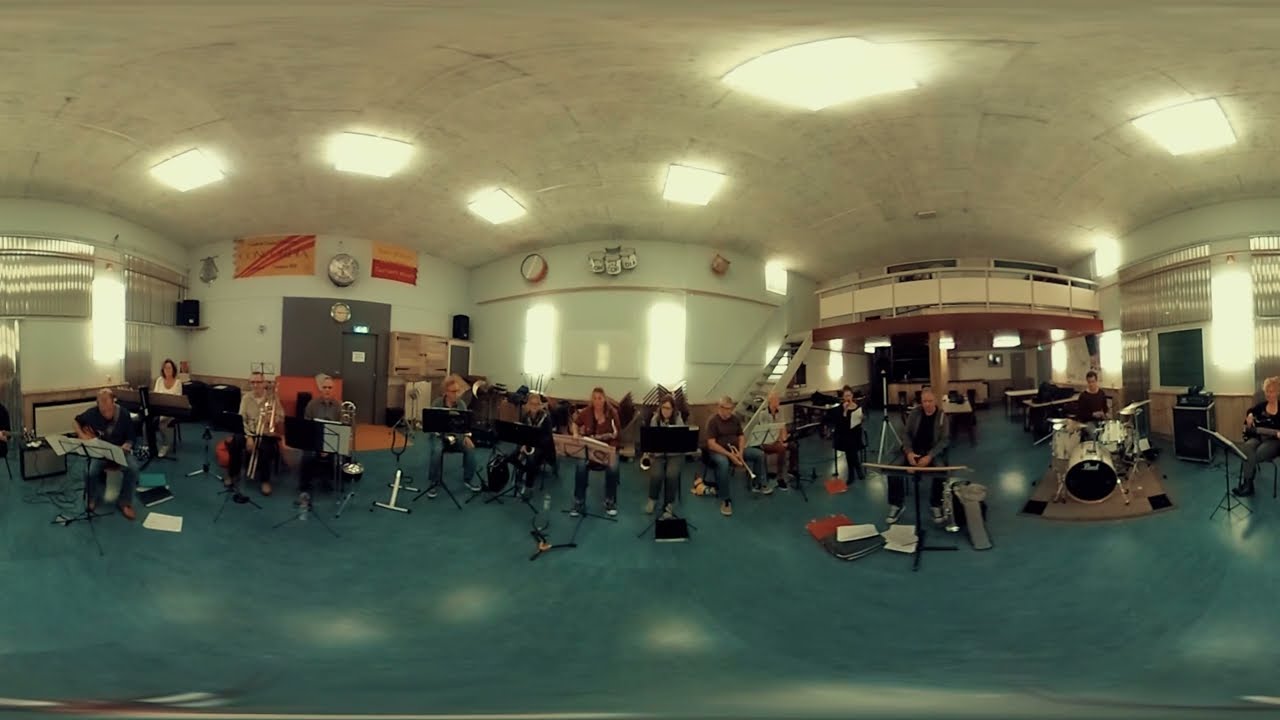The photograph captures an indoor scene of a musical band or symphony performing in a large, likely acoustically designed room, possibly a concert or practice hall. The space features prominently curved, white walls and a curved ceiling, giving it an architectural flair. In the background, there is a large entrance and a balcony to the right, making the room feel expansive. The floor is a dark blue concrete-like surface that reflects the ceiling lights scattered throughout the hall. 

The musicians, all dressed in dark colors except for a woman in a red shirt and blue jeans, are seated on chairs arranged in rows. Each musician has a black stand in front of them containing sheet music. Notable members include a drummer positioned on the right, a man with a keyboard at the center, and a saxophonist. There's a light above a door on the left side, with two indistinguishable red and yellow flags above it.

Decorative banners and round objects hang from the walls, enhancing the space’s aesthetic. The room lacks windows, leaving the time of day indeterminate. The detailed setting combined with the musicians deeply focused on their instruments and sheet music creates a formal and immersive atmosphere.